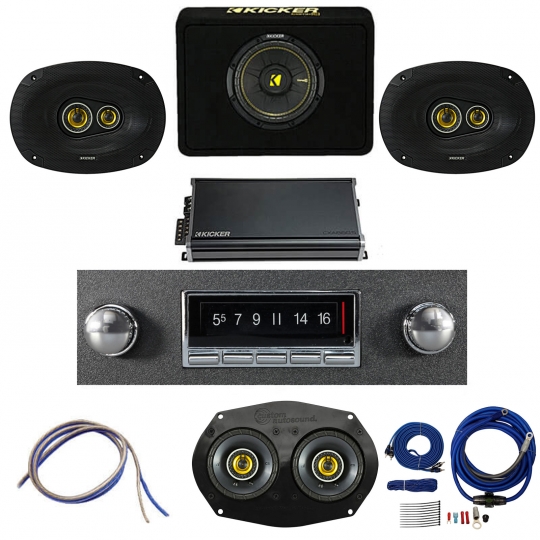The image depicts a collection of Kicker-branded audio equipment, which appears to be showcased for sale, possibly on a site like Amazon. In the upper portion, there are several black speakers with yellow logos and accents clearly marked with the brand "Kicker". Flanking these speakers are elongated, oval-shaped units. Below the speakers is a rectangular metallic amplifier bearing the Kicker logo. The central part of the image features a detailed control panel with various knobs, buttons, and number settings - 5, 7, 9, 11, 14, and 16 prominently visible. At the center bottom, there is a black speaker. Additionally, the lower left section of the image shows neatly spooled white and blue cables, while the lower right contains more audio cables with jack ends and smaller adapters. The overall image is sharply captured in a brightly lit setting, making every element clear and distinct.